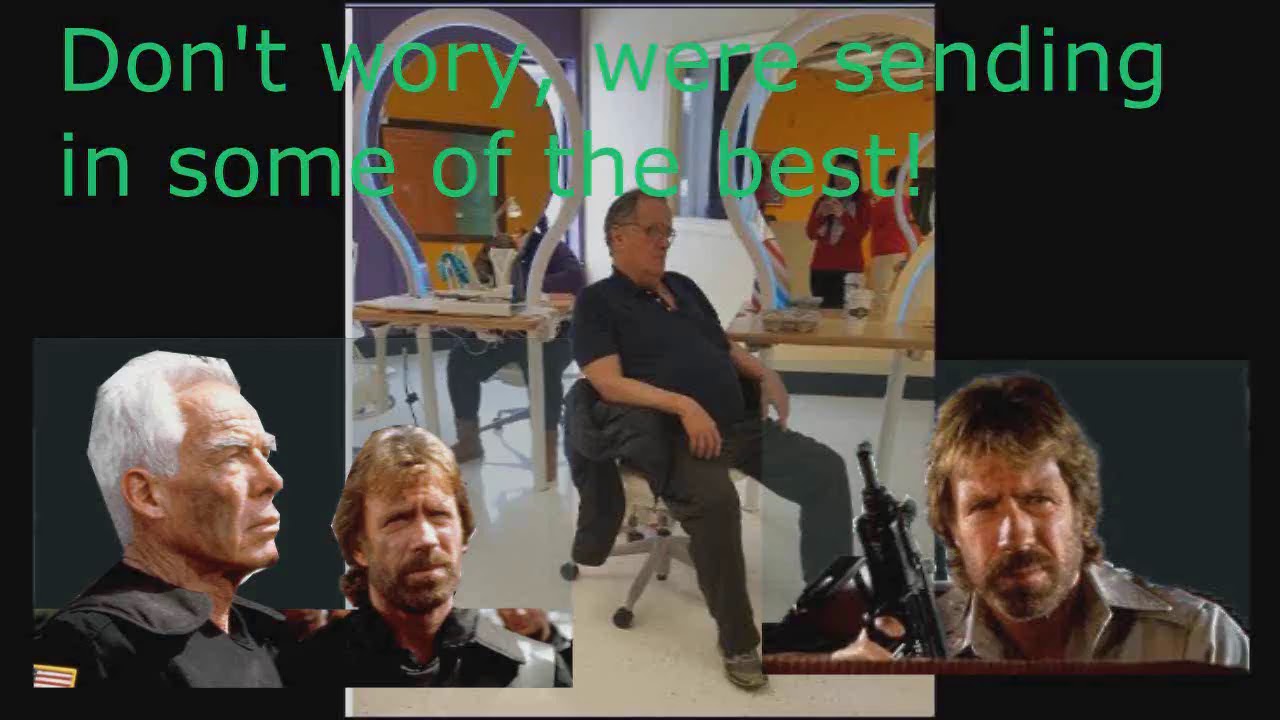In this image, a bespectacled man in a black polo shirt and black pants leans back in a swivel chair in what appears to be a salon or a makeup preparation area. He sits between two vanities, each adorned with rounded mirrors and supported by white legs. His expression suggests weariness, as if he has had enough for the day. Above him, green text reads, "Don't worry, we're sending in some of the best." Three smaller, photoshopped images float around the man: one on the right and two on the left. These images feature Chuck Norris and Lee Marvin. On the right, Chuck Norris is seen holding a machine gun, staring ahead with a suspicious look. On the left, one image shows Chuck Norris with brown, feathered hair and facial hair, while the other depicts an older, white-haired Lee Marvin with prominent white eyebrows.